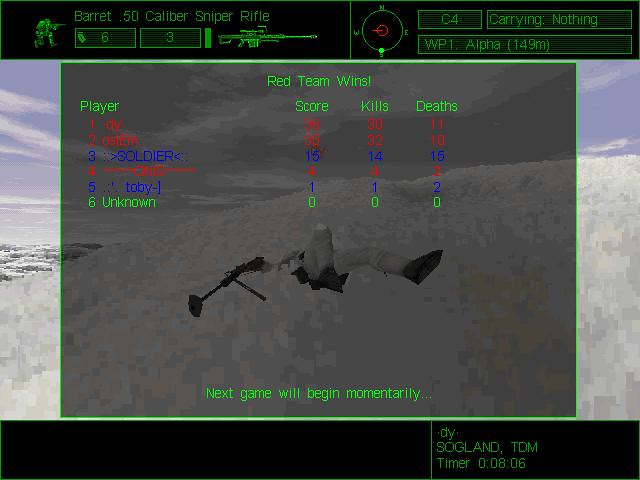The image is a pixelated screenshot from a video game set in a monochrome, possibly black and white, environment with overlaying colored text for instructions and information panels. The primary focus of the scene is a small avatar lying flat on an expansive snowy landscape, indicating the character has been defeated or lost the game. In the center of the screen, a message declares "Red Team Wins," with a comprehensive scoreboard listing players, scores, kills, and deaths in green, red, and blue fonts. The top of the screen features detailed information about the weapon used, a Barrett .50 caliber sniper rifle, and other status indicators such as "Six mags, three bullets," "C4 carrying nothing," and "WP1 Alpha 149M." Above this, there are two boxes: one displaying a tiny animated soldier figurine holding a gun, and the other showing a compass pointing west. On the bottom black bar, a timer reads "T.D.M. TIMER 008:06," possibly indicating the game's duration. Finally, a message at the bottom center of the screen announces, "Next game will begin momentarily," signifying a brief pause before the next round. The entire scene is framed with black bars at the top and bottom, adding to the encapsulated arcade-style aesthetic of the image.